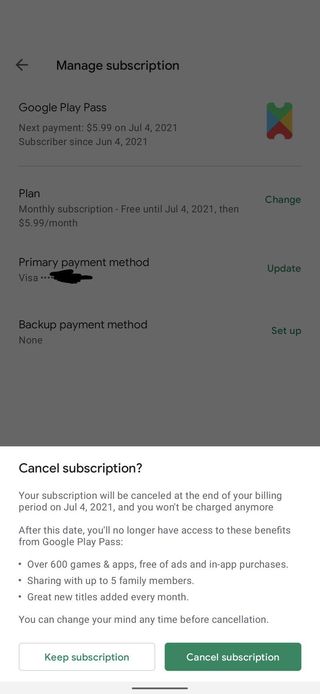The image displays a mobile phone screen showcasing a subscription management interface for Google Play Pass, which has been grayed out due to the initiation of a subscription cancellation process. The primary section, a grayed-out rectangle, includes the following detailed information:

- **Header**: A left arrow icon indicating navigation, followed by the text "Manage Subscription".
- **Subscription Details**: The label "Google Play Pass" with the next payment amount of $5.99 scheduled for July 4th, 2021, and the subscriber's start date of June 4th, 2021.
- **Graphics**: To the right, an icon resembling a ticket colored with green (top), red (bottom), yellow (right), and blue (left). A faint line extends from the 'G' in "Google" to the end of the ticket.
- **Plan Description**: Text stating "Monthly Subscription, free until July 4th, 2021, then $5.99 a month". Adjacent to this text is a green "Change" button.
- **Payment Methods**: The primary payment method is listed as "Visa" with card details protected by asterisks. Next to this is an "Update" button. Additionally, there is a "Backup Payment Method" which is currently set to "None". There is an option to "Setup" a backup method beside it.
- **Cancellation Confirmation**: Below the grayed-out box, the text confirms that the subscription will be canceled at the end of the billing period on July 4th, 2021, and no further charges will be made. It informs the user that after this date, the benefits of Google Play Pass will be lost.
- **Benefits Listed**: Three bullet points highlight the benefits of the subscription—access to over 600 games and apps free of ads and in-app purchases, ability to share with up to five family members, and the addition of great new titles monthly.
- **Action Buttons**: At the bottom, there are two buttons— "Keep Subscription" in green writing on a white button on the left and "Cancel Subscription" in white writing on a green button on the right.
- **Additional Element**: A gray rectangle in the middle featuring a black line.

This detailed depiction is framed within the context of a mobile user interface where a subscription service is actively being managed and canceled.